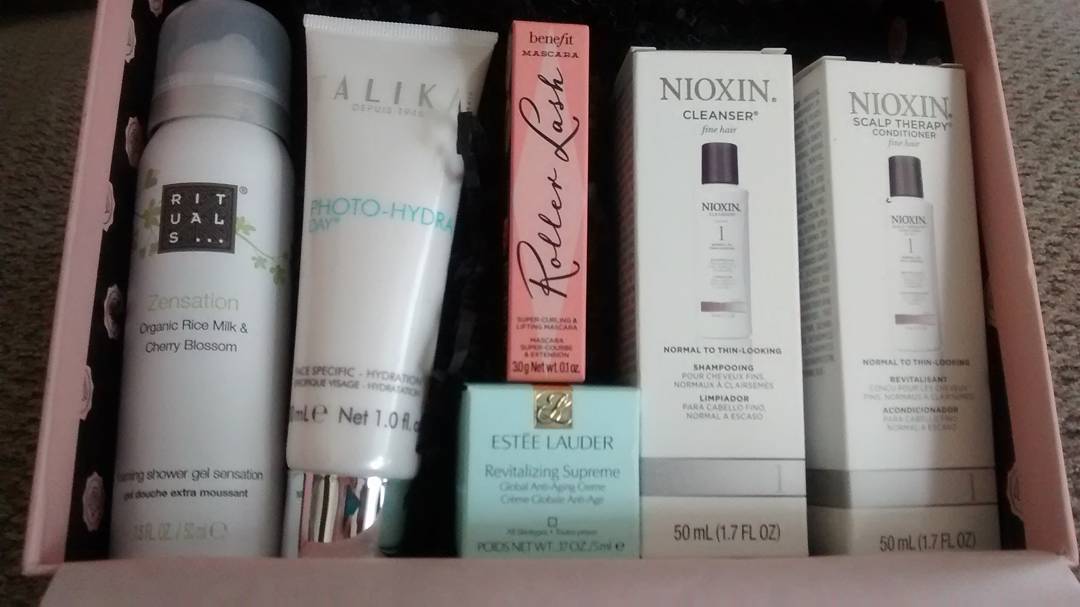The image showcases a meticulously arranged close-up of a facial care product box, with the visible interior predominantly pink, transitioning to black at the bottom. 

On the left side, there is a cylindrical, white bottle with a clear cap. The bottle is branded with the name "RITUALS" in a staggered format – "RIT" on the first line, "UAL" on the second, and an obscured "S..." on the third. An elegant ivy plant design weaves from the right side, curving under the RITUALS logo and resuming on the other side. The product is identified as "Zensation," featuring Organic Rice Milk and Cherry Blossom, and it is categorized as a shower gel.

Adjacent to it is another product whose top letters are not completely visible. The larger discernible text reads "ALIK," and further down it is labeled "PHOTOHYDRA," followed by some smaller, indistinct text at the bottom.

Centrally placed is a small, elongated box labeled "ROLLER LASH." Below that sits a green square box branded with "Estée Lauder."

On the right, there are two boxes from Nioxin. The first box is labeled "Cleanser," while the second one is "Scalp Therapy."